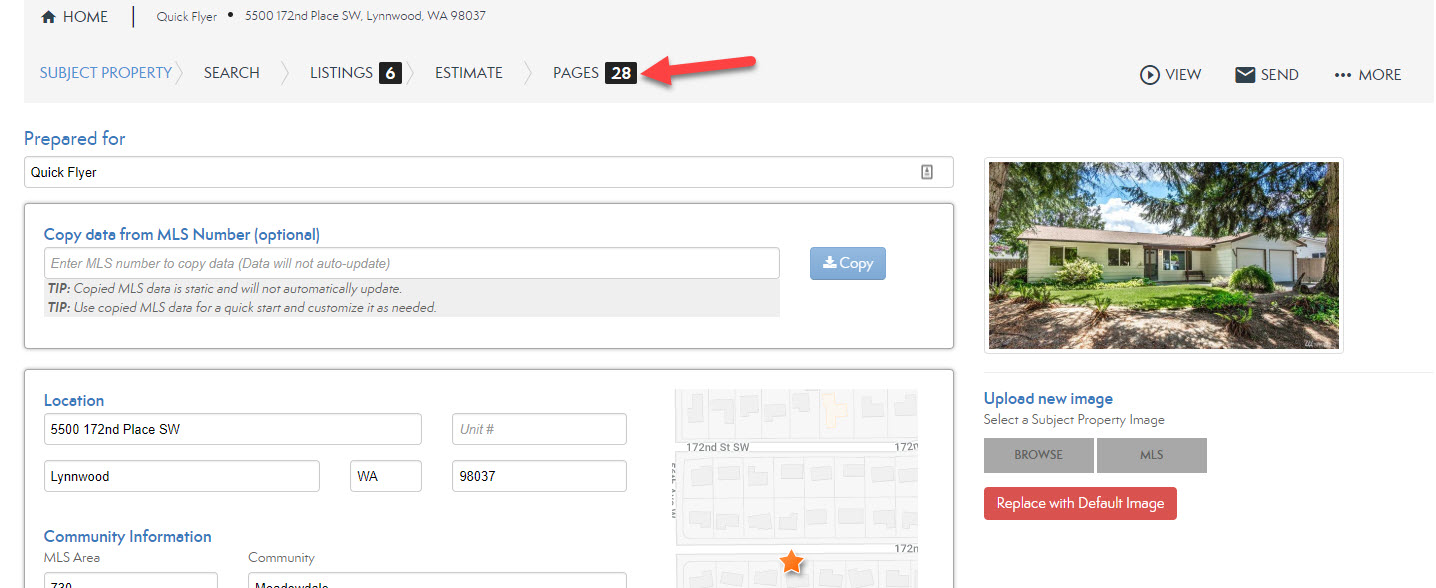A screenshot is displayed against a white background, detailing a real estate website interface. In the upper left corner, the website header reads "Home" and "Quick Flyer." Below, the address "5500 172nd Place, Southwest, Lynnwood, Washington, 98037" is prominently featured. The phrase "Subject Property" is highlighted in blue text.

A black box with the number "6" appears next to options for "Search," "Listings," and there are details about the property estimation, indicating that it spans "28 pages." The interface also includes buttons labeled "View," "Send," and "More."

The document is titled "Prepared for: Quick Flyer," and there is an option to "Copy Date from MLS Number" with a corresponding "Copy" button. Below this, a tip informs users that "Copied MLS data is static and will not automatically update," and advises to "use copied MLS data for a quick start and customize as needed."

Further down, the property location is reiterated: "5500 172nd Place, Southwest, Lynnwood, Washington, 98037." To the right, a small map marks the house's location with a star icon.